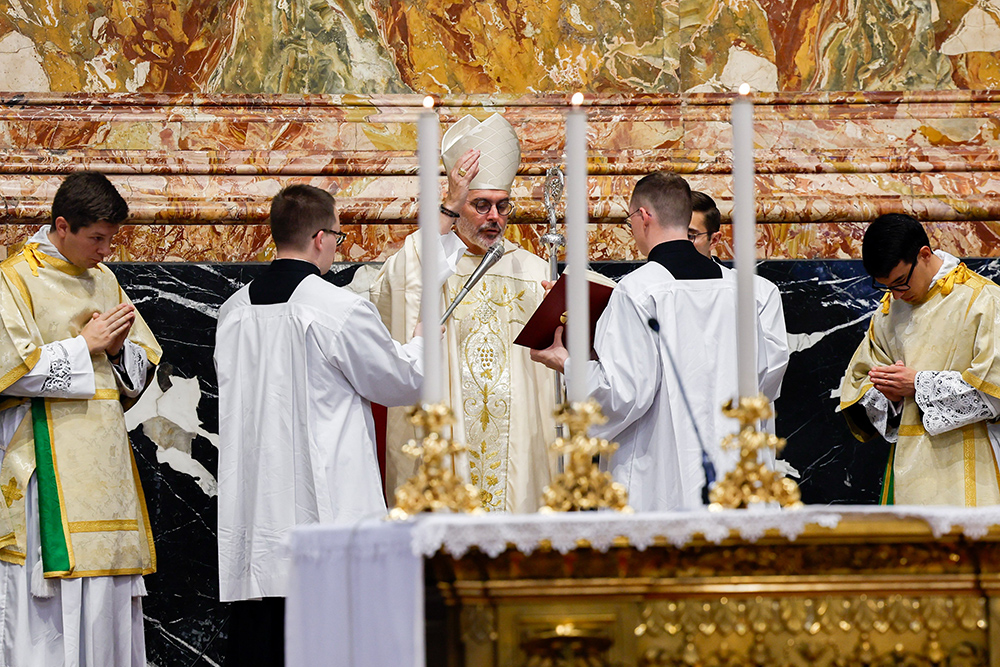This detailed photograph captures a Catholic church mass, featuring an ornately decorated marble interior vibrant with hues of orange, red, green, and mustard yellow. Central to the scene is a priest adorned in white robes with gold embroidery and a distinctive, white, pope-like hat. He stands behind a golden altar, upon which rest three large, white pillar candles in elegant gold candlestick holders, their light slightly blurred in the foreground. The priest is depicted reading from a book held by an altar boy while raising his right hand in a gesture, and gripping a silver staff with a curled top in his left hand. Flanked by several altar boys in white robes, two assist directly, one holding a microphone and another glimpsed just enough to show his head and shoulder. Two additional altar boys, donned in robes with gold details, stand at the far left and right, heads bowed and hands clasped in prayer, facing the priest in solemn reverence. The overall scene emanates a sense of ceremonial grandeur and spiritual focus.